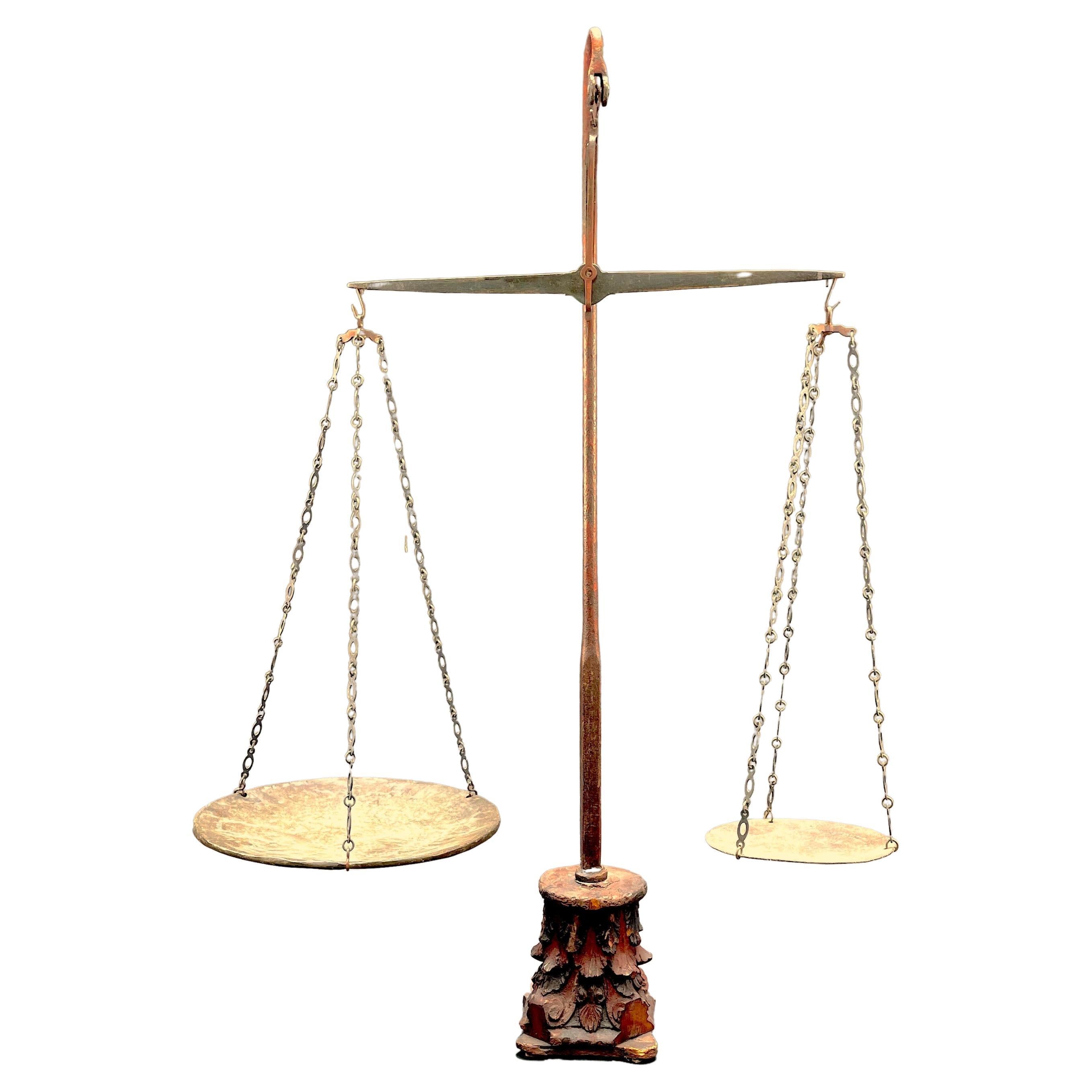This photograph features an old-fashioned, ornate weighing scale reminiscent of the Libra sign, often symbolizing justice. The scale boasts a meticulously carved wooden base adorned with leaf-like or possibly fish scale patterns. Rising from this decorative base is a vertically oriented pole, which transitions into a crossbar made of a grayish metal at the top. The crossbar supports two circular metal plates, each suspended by three golden chains from hooks on either end. The left plate is notably larger in diameter than the right, although the scale remains balanced, suggesting an equal distribution of weight. The metal plates have a gold hue, and the entire setup is centered against a stark white background that emphasizes its antique and symbolic nature.